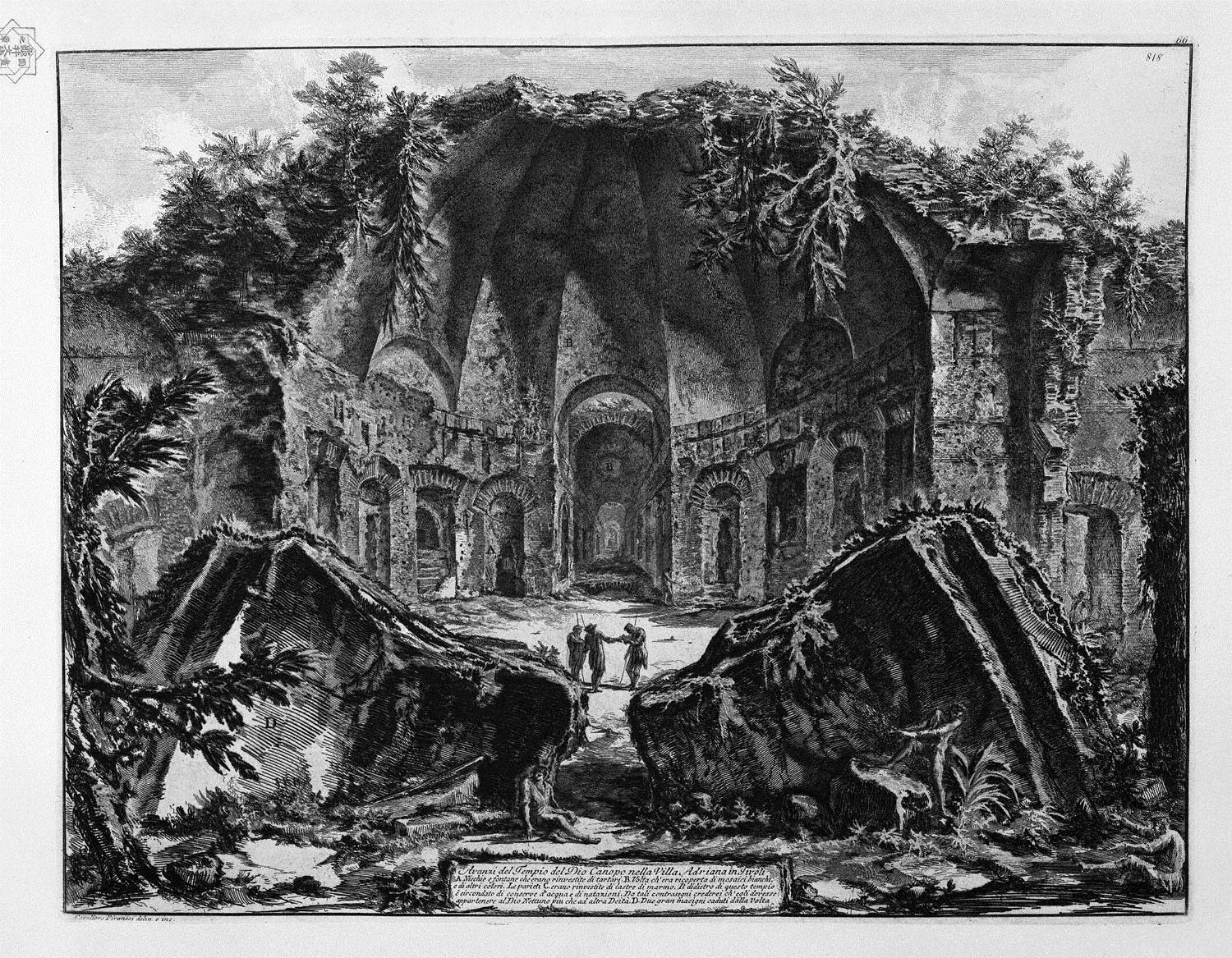This black-and-white illustration, possibly a lithograph print or pen-and-ink drawing, depicts a dilapidated structure that resembles a cathedral or castle, richly detailed and evocative of an old newspaper or vintage magazine style. The central feature is an arched doorway that leads to a wide-open, domed section, partially destroyed and overrun with foliage. Trees and bushes spill over into the structure, emphasizing its state of neglect and overgrowth. Flanking the main doorway are several smaller arched doors. The building appears severely damaged, with two sides having collapsed at angles. In the foreground, three figures stand in front of this central, arched ruin, while another individual sits in the lower right corner, reaching out towards the structure. Additional text is present at the bottom of the image, though it remains too small to decipher. This meticulous and intricate artwork captures the haunting beauty of decay.